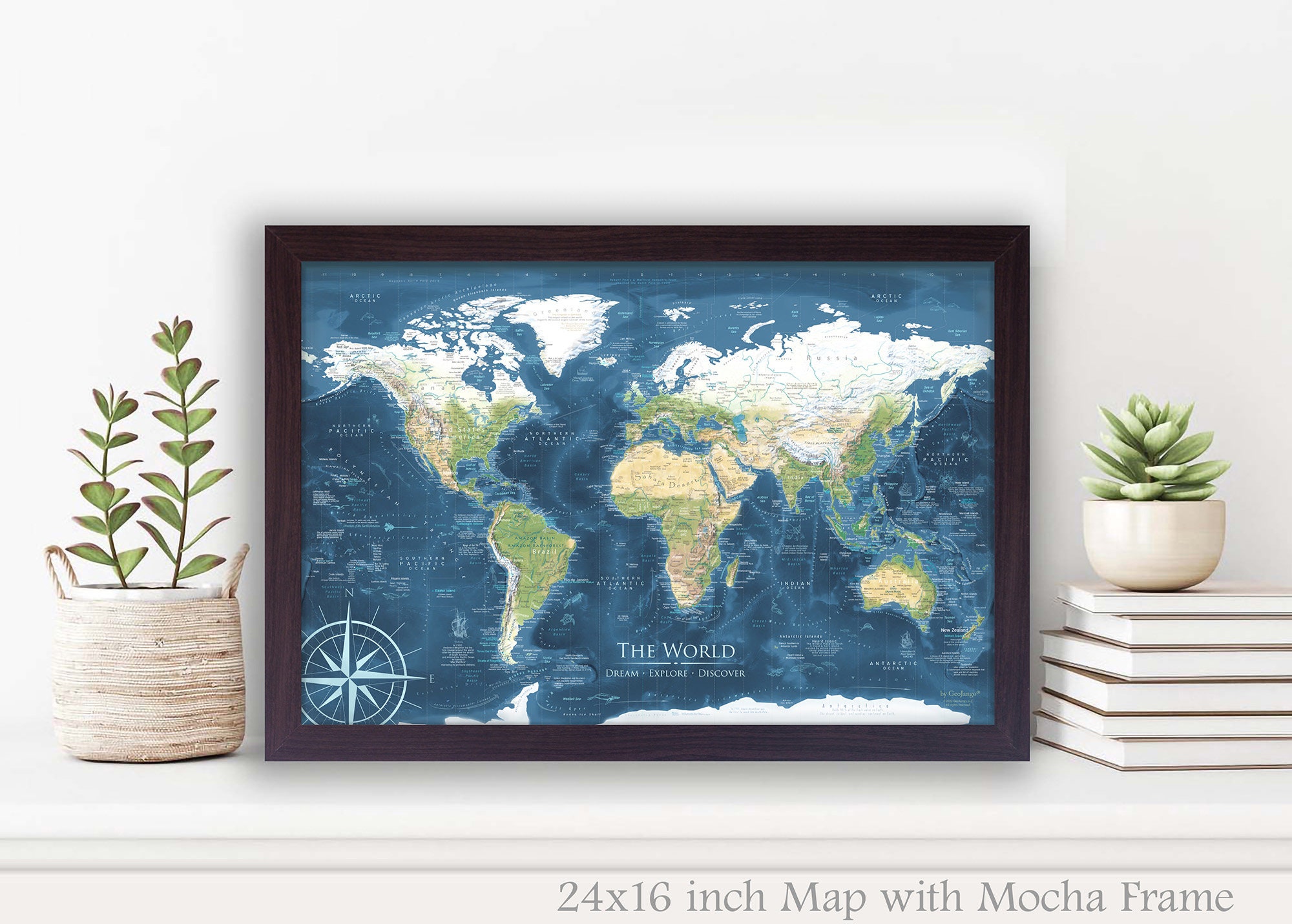This is a detailed product photo of a framed Mercator-style world map, measuring 24 by 16 inches with a mocha frame. The map is positioned atop a white table against a white background, creating a clean, uncluttered look. It features typical color coding: the northern regions are white to represent snowy, cold areas; green hues indicate forested regions; and brown marks mountainous and desert areas. The central areas of Africa and Europe are prominently displayed, with North and South America on the left and Asia on the right. The map includes picturesque ocean hues and a large compass in the bottom left corner. On either side of the map are potted plants; one larger plant with brown stripes that sits directly on the table, and another smaller plant that rests atop a stack of six books on the right side. The scene appears carefully staged, possibly photoshopped, for an enhanced aesthetic. At the bottom of the map, text reads, "The World: Dream, Explore, and Discover."